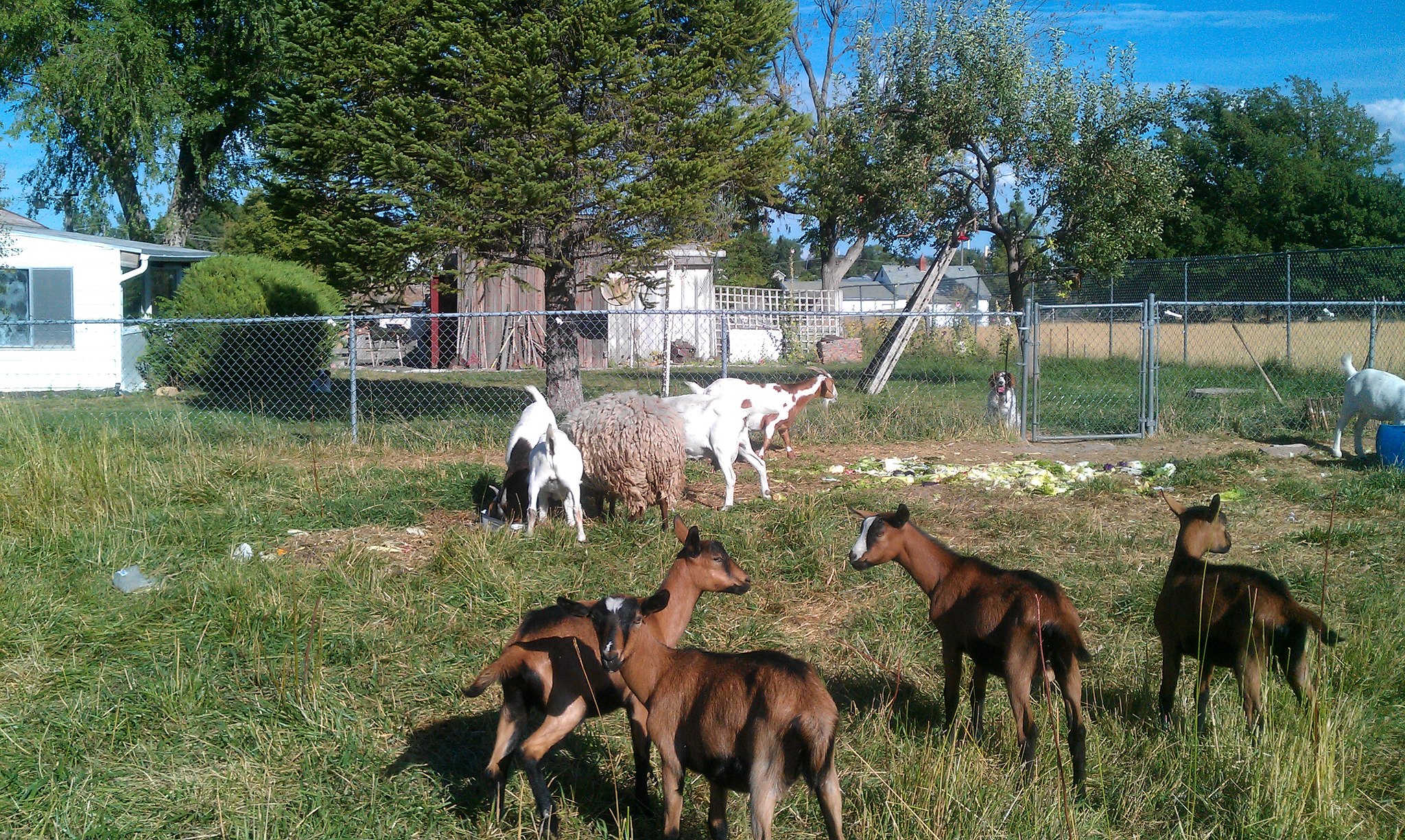In this vibrant outdoor daytime color photograph, the focus is on a group of farmyard animals enclosed within a stainless steel chain-link fence that spans horizontally across the middle of the image, featuring a gate on the right side. The pen is shared by several brown goats in the foreground and a single woolly sheep in the center, with its coat facing away from the viewer. The grassy area within the pen is overgrown, interspersed with patches of bare soil and brown grass. In the lush setting, a total of around four goats are clearly visible in the foreground, accompanied by a shaggy, off-color brown sheep to the left, and more goats and sheep scattered in the background.

A white-bodied dog with brown ears is positioned just outside the fence, slightly right of center, attentively watching the animals. On the left side of the image, behind the fence, the white siding of a house with a couple of visible window panes can be seen. The periphery of the image is framed by tall green trees and bushes, underlining the blue sky with wisps of white and grey clouds filtering through the canopy. This detailed scene captures the peaceful coexistence of farmyard life under a bright, beautiful sky.